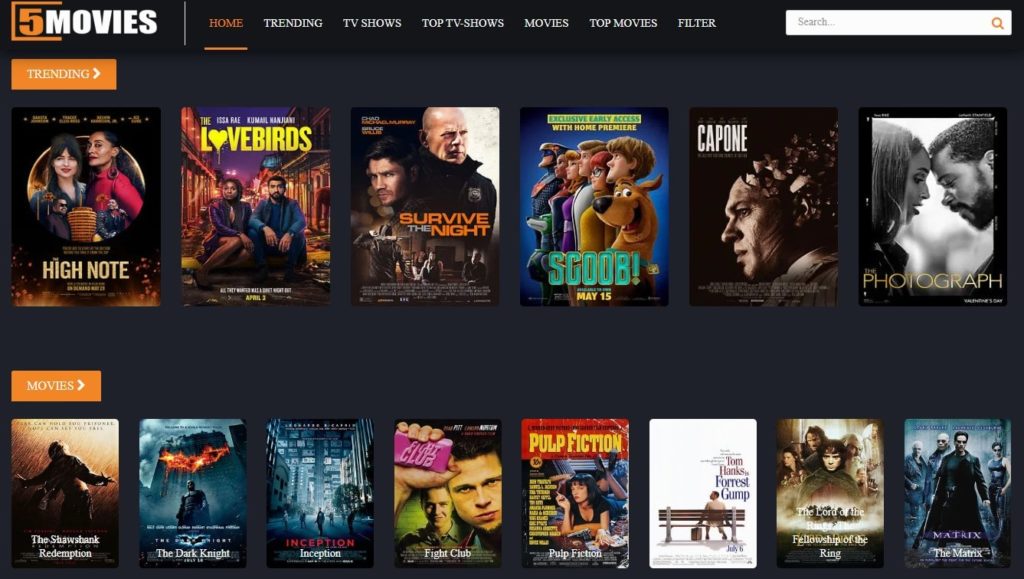The homepage of 5 Movies features a sleek design with the number '5' displayed in vibrant orange alongside the word 'Movies' in clean white typography. The interface offers an array of categories including Home, Trending, TV Shows, Top TV Shows, Movies, Top Movies, and Filter, ensuring easy navigation for users. Prominently placed is a white search box accented with an orange magnifying glass icon, allowing for quick searches.

Scrolling through the Trending section, various popular movies are showcased. "High Note" stands out with a diverse cast around a towering building. "The Lovebirds" features a couple seated together on a city street, capturing a moment of intimacy. "Survive the Night" displays two men in black uniforms, suggesting a tense, confrontational scenario. "Scoob" boasts an 'Exclusive Early Access with Home Premiere,' presenting a cartoon family and their dog in a whimsical lineup. "Capone" portrays a troubled individual with chaotic imagery emanating from their head, hinting at psychological depth.

Additionally, a classic black-and-white photograph captures a poignant moment between a man and a woman, their foreheads touching as they gaze into each other's eyes. The homepage also celebrates classic cinema with movie posters for enduring favorites like "Forrest Gump," "Fight Club," "Pulp Fiction," and "Inception," among others, offering a rich mix of contemporary hits and timeless treasures.